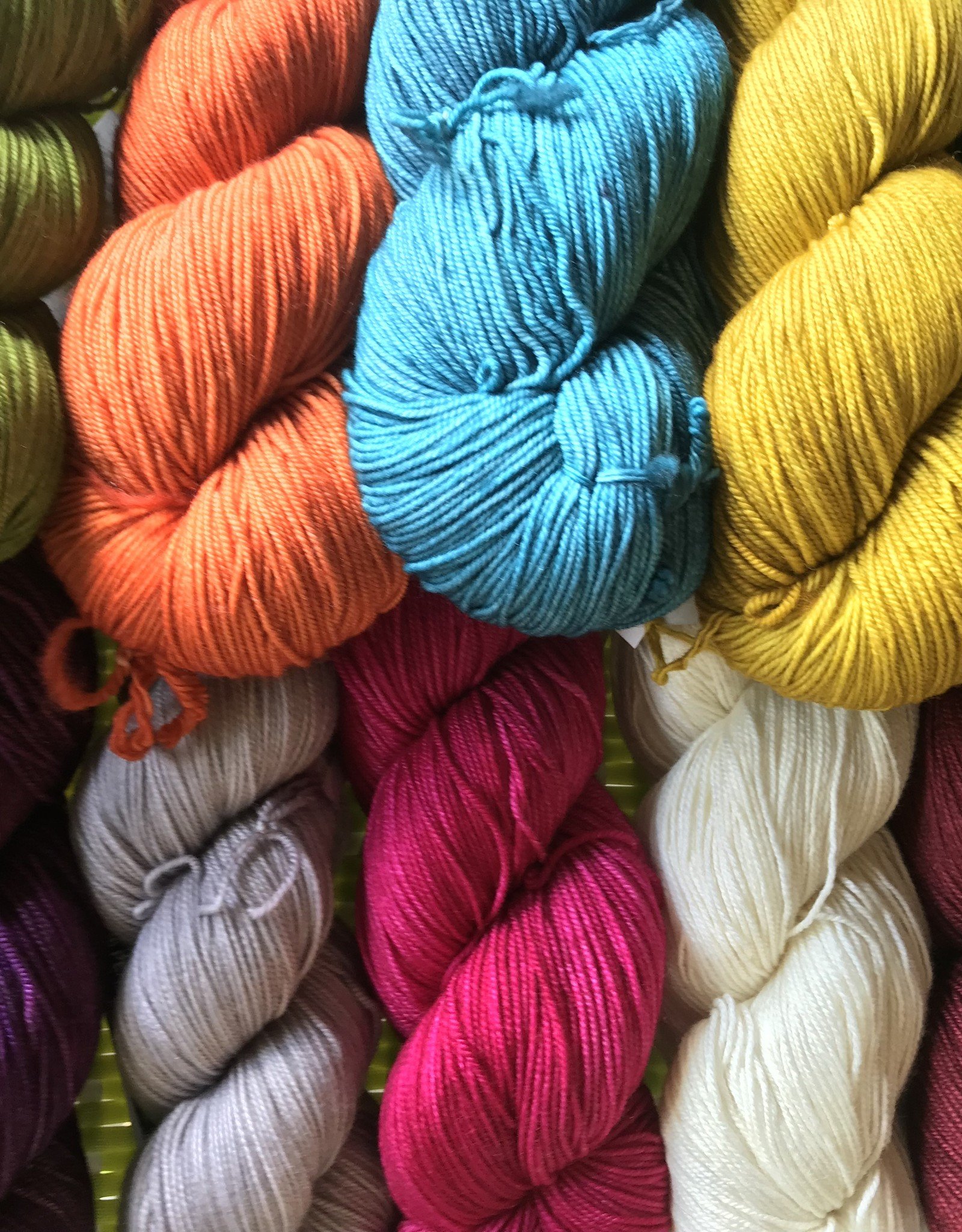This image is an up-close shot of a collection of brightly colored yarn skeins, intricately arranged and tied together in three central places. The yarns appear smooth and vibrant, featuring a mix of colors such as light green, orange, light blue, yellow, purple, gray, pink, white, and fuchsia. They are coiled up, with four prominent coils visible at the top and four at the bottom, filling the frame. This arrangement creates a visually appealing pile that one might find in a fabric store or a craft storage area. The background, which is likely a greenish surface, is mostly obscured by the densely packed and vibrant yarn. The image showcases the yarns' rich, engaging colors, drawing attention to their smooth texture and the orderly yet creative way they are displayed.